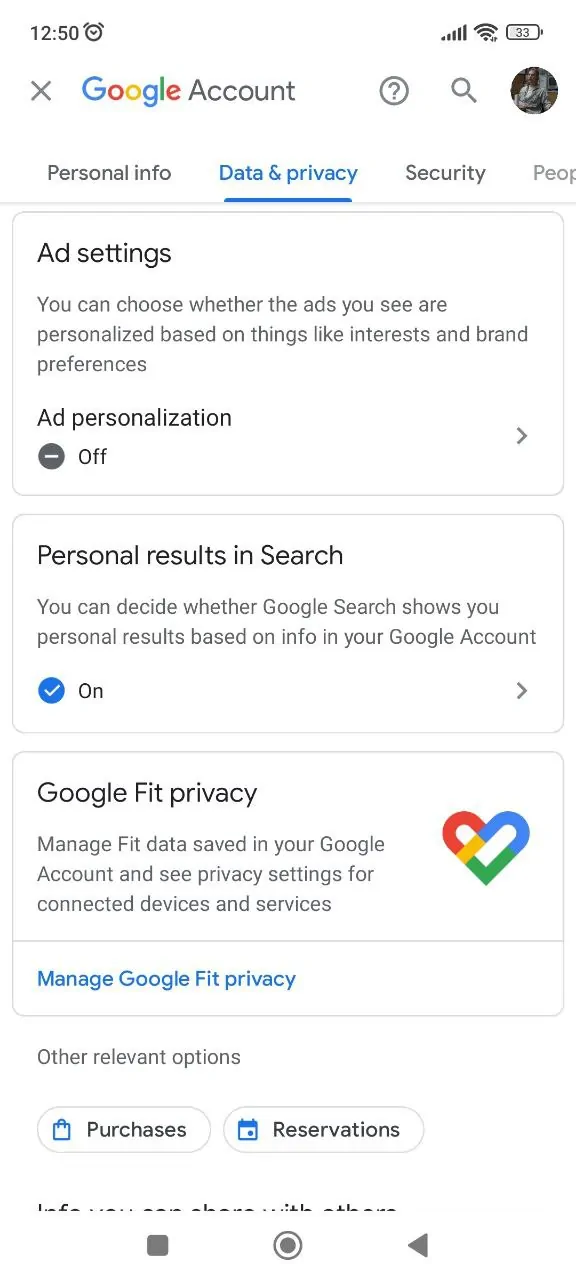The image is a screenshot of a Google Account settings page. The top left corner displays the time as 12:50, with a black alarm icon beside it. The battery life indicator shows 33%, and the device has a good network connection. 

At the top, the words "Google Account" are prominently displayed in a colorful Google logo, with "Google" in green, red, yellow, and blue. Next to this text is a small, dark, and barely visible profile image of an individual, alongside a search icon and a circular icon with a question mark inside.

Below the header, there is a navigation bar with three sections: "Personal info," "Data and privacy" (highlighted in blue), and "Security" (in gray). The fourth section label is partially obscured but appears to start with "People."

A section titled "Ad settings" follows, where it explains that users can choose whether the ads they see are personalized based on interests and brand preferences. The text "Ad personalization" is displayed in dark gray, accompanied by a circle with a white line, indicating that the feature is off. An arrow pointing to the right suggests additional options.

Next is a section on "Personal results in search." It explains that users can decide whether Google Search shows personal results based on their account information. A blue circle with a checkmark indicates this feature is enabled.

The third section is "Google Fit Privacy," which allows users to manage Fit data saved in their Google Account and review privacy settings for connected devices and services. This section features a colorful Google Fit heart icon in blue, red, yellow, and green. The phrase "Manage Google Fit Privacy" is highlighted in blue, indicating it's clickable.

At the bottom of the screenshot, there's a reference to other relevant options, such as "Purchases" and "Reservations."